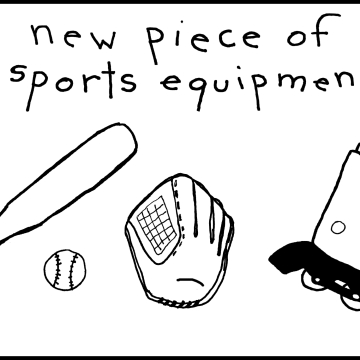The black and white illustration is a hand-drawn image, likely created on paper or digitally on a computer, such as with Microsoft Paint. The image is framed by two horizontal black lines, one at the top and one at the bottom. Between these lines, at the top, there is handwritten text that reads, "New Piece of Sports Equipment," although the T in "Equipment" is partially or entirely cut off. Below the text, various sports items are depicted. On the left, there's the cut-off tip of a baseball bat followed by a roughly sketched baseball. In the center, there is a baseball glove featuring a rectangular grid pattern. To the right, there is an illustration that appears to be a pair of eyes with a thick black line resembling a unibrow over them; a perpendicular line extends outward, indicating it could be the rim of glasses. Some descriptions suggest this may be a simplified sketch of a roller blade, showing part of the boot, two wheels, and a braking pad. The entire layout suggests a casual, artistic style with imperfect, hand-drawn quality.